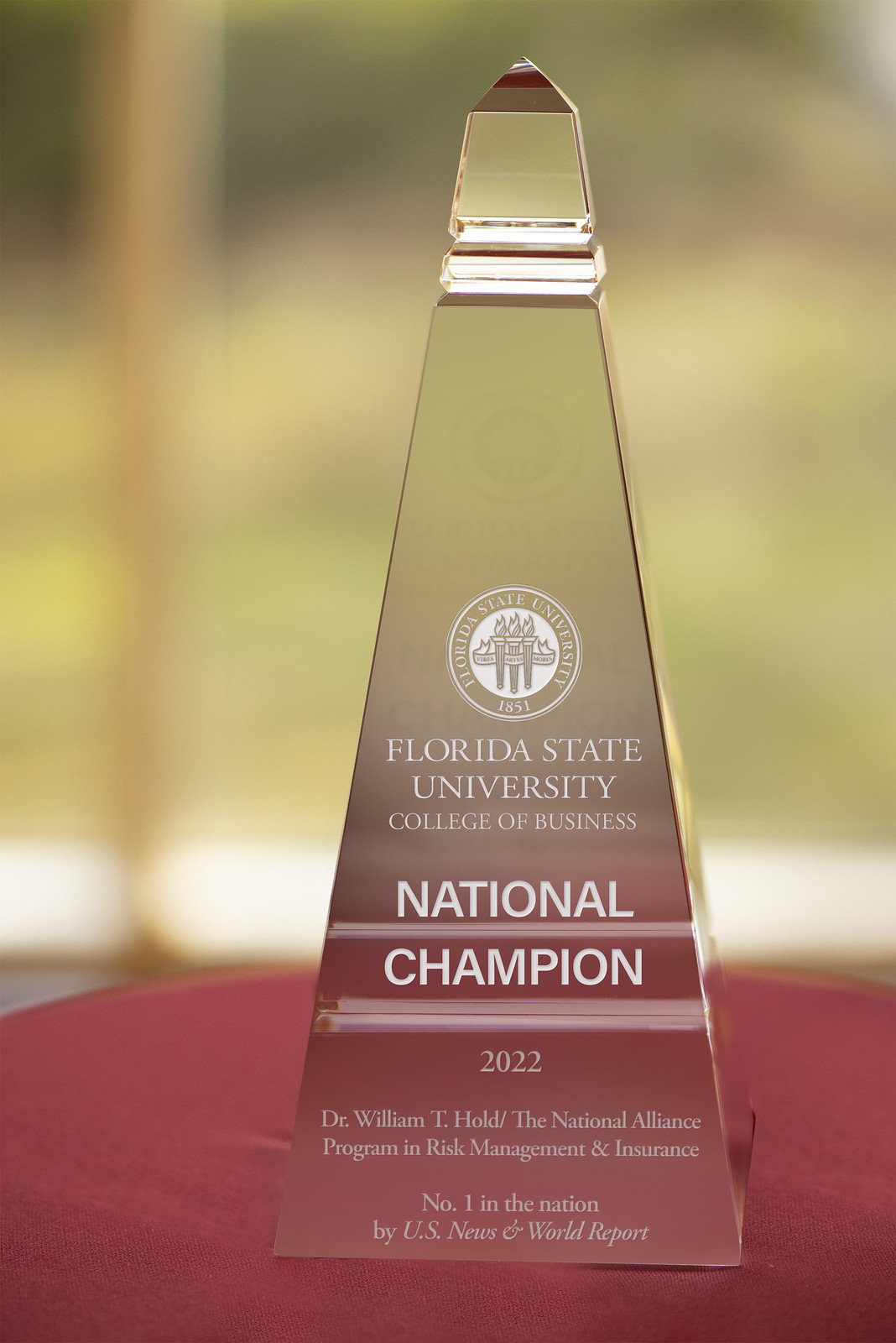The photograph features a tall, obelisk-shaped trophy resembling a stretched pyramid. Made from a reflective glass or metal material, the trophy has intricate etchings in white text and symbols. Centrally positioned on the trophy is a circular logo containing three torches, encircled by the words "Florida State University, 1851." Below the logo is an inscription that reads: "Florida State University College of Business National Champion, 2022. Dr. William T. Hold, The National Alliance Program in Risk Management and Insurance, Number One in the Nation by US News and World Report." The trophy is positioned on a round table draped in a reddish-burgundy fabric, while the background of the image is blurred, emphasizing the award.